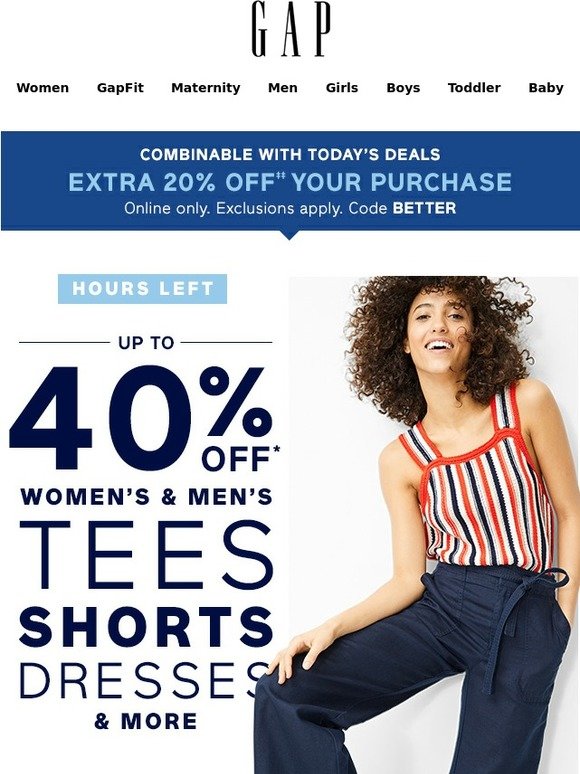This image is an advertisement for The Gap, presented with a clean, minimalistic design typical of the brand's aesthetic. Set against a white background, the top of the image prominently features The Gap's name and logo, which consists of the letters "G-A-P" in capitalized, slender font. Below the logo, there is a horizontal list of categories in black text, possibly indicating clickable links: "Women," "GapFit," "Maternity," "Men," "Girls," "Boys," "Toddler," and "Baby." 

A bit further down is a distinctive blue rectangle banner, containing a promotional message in white and light blue text: "Combinable with Today's Deals, Extra 20% Off Your Purchase, Online Only, Exclusion Apply, Code: BETTER."

The main visual is of a young woman with curly brown hair, modeling an outfit consisting of a striped shirt in shades of orange, white, and brown with over-the-shoulder straps, paired with blue slacks. Adjacent to this image, text highlights the central offer of the ad: "40% off women's and men's tees, short dresses, and more."

The layout and style suggest that this could be a screenshot from The Gap's mobile or tablet site, or an embedded ad on a webpage.